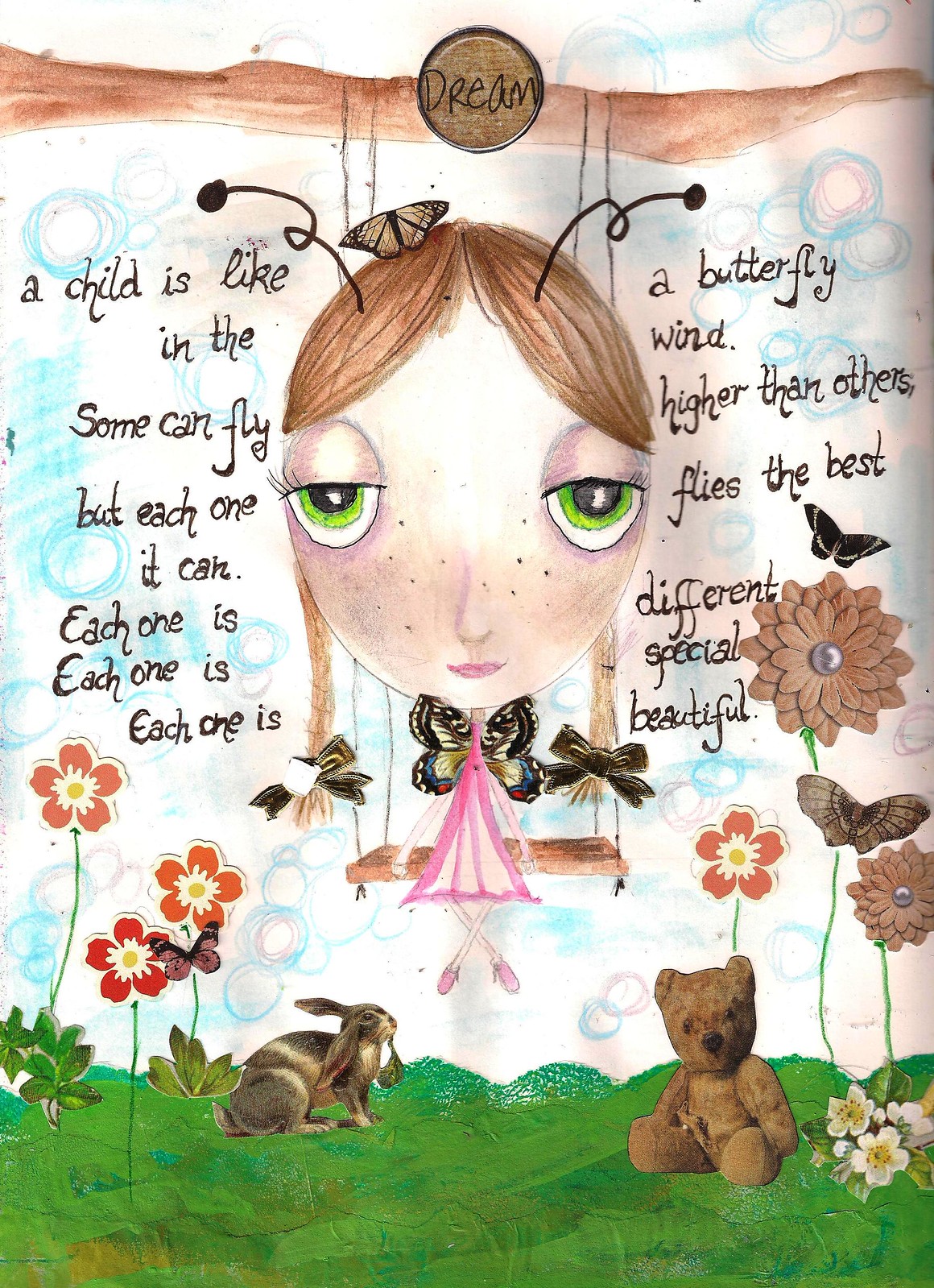The image is an intricate painting resembling a book cover, featuring a whimsical scene centered around an oversized-headed little girl with brown hair, parted in the middle. Her hair is adorned with ribbons and she has antennas with bulbs on the ends, accentuating her insect-like appearance. The girl’s captivating green eyes, complete with spindly eyelashes and freckles, add to her charmingly surreal aura. She wears a pink dress and butterfly wings on her back, as she sits with crossed legs on a swing that hovers over a lush, grassy hill. 

At the top of the painting, faded blue and red child-like scribbles and circles adorn the background, along with a prominent brownish-red streak running horizontally. A butterfly perches on the girl’s head, contributing to the fantastical theme, while the bottom of the image features a serene garden scene. Here, a rabbit and a teddy bear rest among vibrant flowers, some orange and brown, blooming towards the sky. The entire artwork seems to be floating in an imaginative landscape.

Flanking the girl's figure in elegant calligraphic text are the touching words: "A child is like a butterfly in the wind. Some can fly higher than others, but each one flies the best it can. Each one is different, each one is special, each one is beautiful." The combination of these elements paints a dreamy, yet detailed portrayal of innocence and individuality.